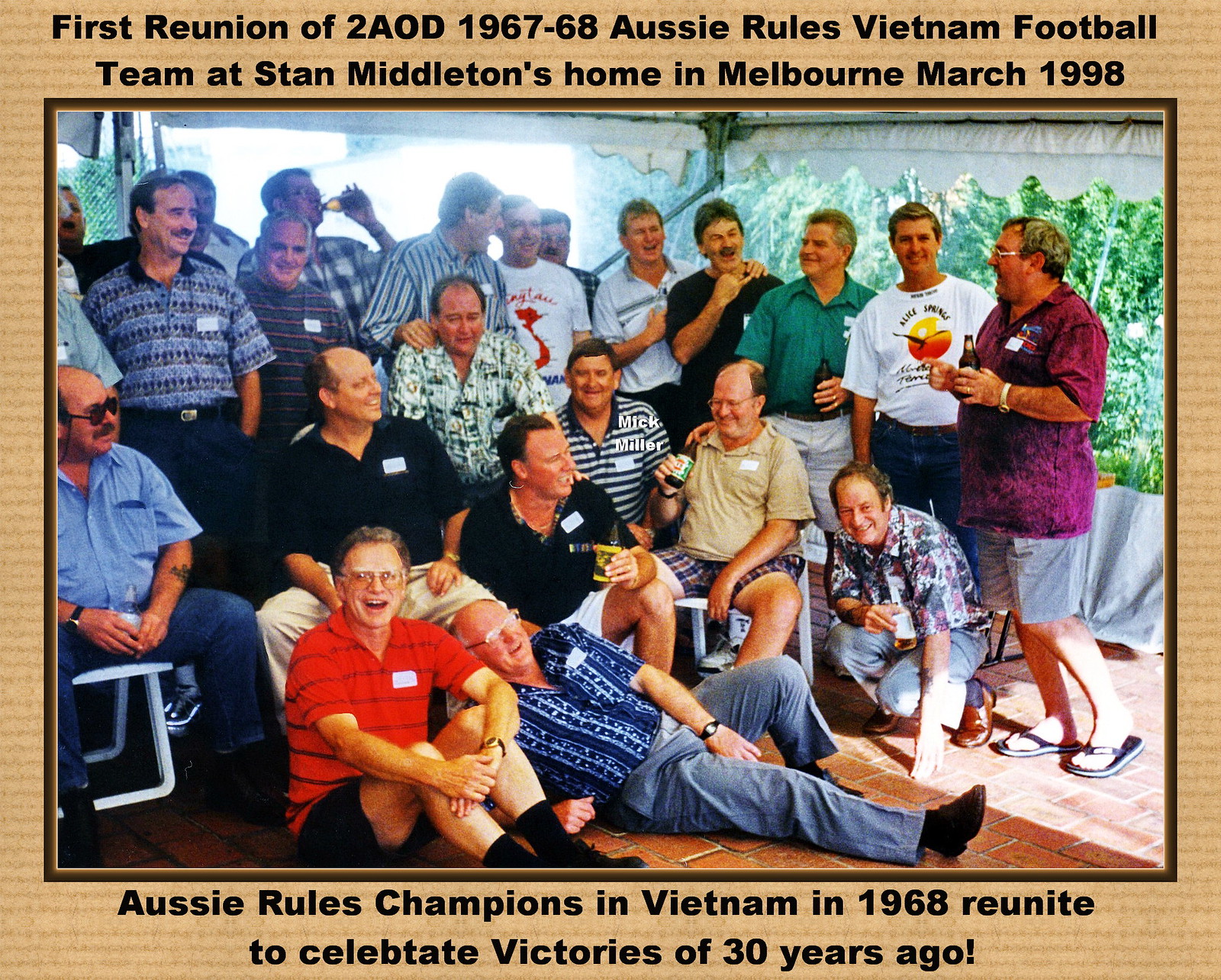This framed photograph captures a joyous moment of reunion for the 2AOD, 1967-68 Aussie Rules Vietnam football team at Stan Middleton's home in Melbourne, March 1998. The tan border with black lettering at the top reads, "First Reunion of 2AOD, 1967-68, Aussie Rules Vietnam Football Team at Stan Middleton's Home in Melbourne, March 1998." At the bottom, it states, "Aussie Rules champions in Vietnam in 1968 reunite to celebrate victories of 30 years ago."

In the center of the image, a large, cheerful group of men poses for the camera. Some men stand while others sit, with one lying on the floor and another sitting on the floor. The setting appears to be an enclosed balcony, evident from the plastic tent-like material in the background through which greenery is visible. The men, many of whom are holding and drinking beers, display big smiles, reflecting their happiness and camaraderie. The image is bathed in a variety of colors, including tan, black, green, yellow, orange, pink, purple, red, blue, and light blue, suggesting celebration and vivid memories of their shared past. The photograph captures not just a reunion, but a celebration of enduring friendship and shared victories, all framed by a warm afternoon gathering.